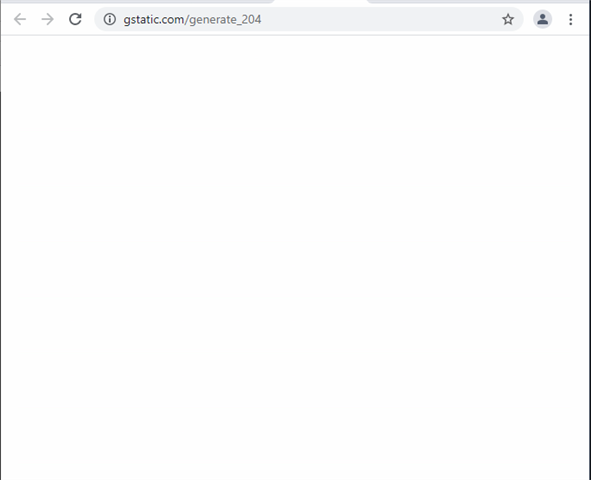The page is predominantly blank with a white background. At the top, there's a navigation and address bar. On the far left, a grey left-pointing arrow is followed by a similar grey right-pointing arrow. Next is a darker circular arrow, which likely indicates a refresh function. The address bar, situated in the center, features a grey encircled lowercase "i" icon on its left side, followed by the URL "gstatic.com/generate_204" displayed in grey text. Towards the right end of the bar, there's a grey outline of a five-pointed star, possibly for bookmarking. Further to the right, there's a grey circular profile icon with a simplistic human figure depicted in darker grey. Adjacent to this, on the far right, are three vertically aligned grey dots, indicating a menu or more options button. The main content section of the page below is essentially empty, maintaining the white background.